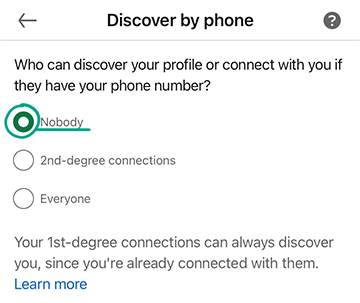A detailed view of a settings screen, specifically focusing on the "Discover by phone" option. The text prompts users to control who can find their profile using their phone number. It reads, “Who can discover your profile or connect with you if they have your phone number?” Options include "Nobody" (currently selected and highlighted), "Second degree connections," and "Everyone." An informative note clarifies that first-degree connections can always discover you since you are already connected. There's also a "Learn more" link for additional information.

As part of what appears to be a tutorial, a pencil has been used to circle the "Nobody" button and emphasize it with an underline. This annotation suggests that clicking "Nobody" will ensure that only your current contacts can reach you, preventing strangers from discovering your profile using your phone number. The visual aids imply that someone is guiding another person on configuring their discovery settings for enhanced privacy.